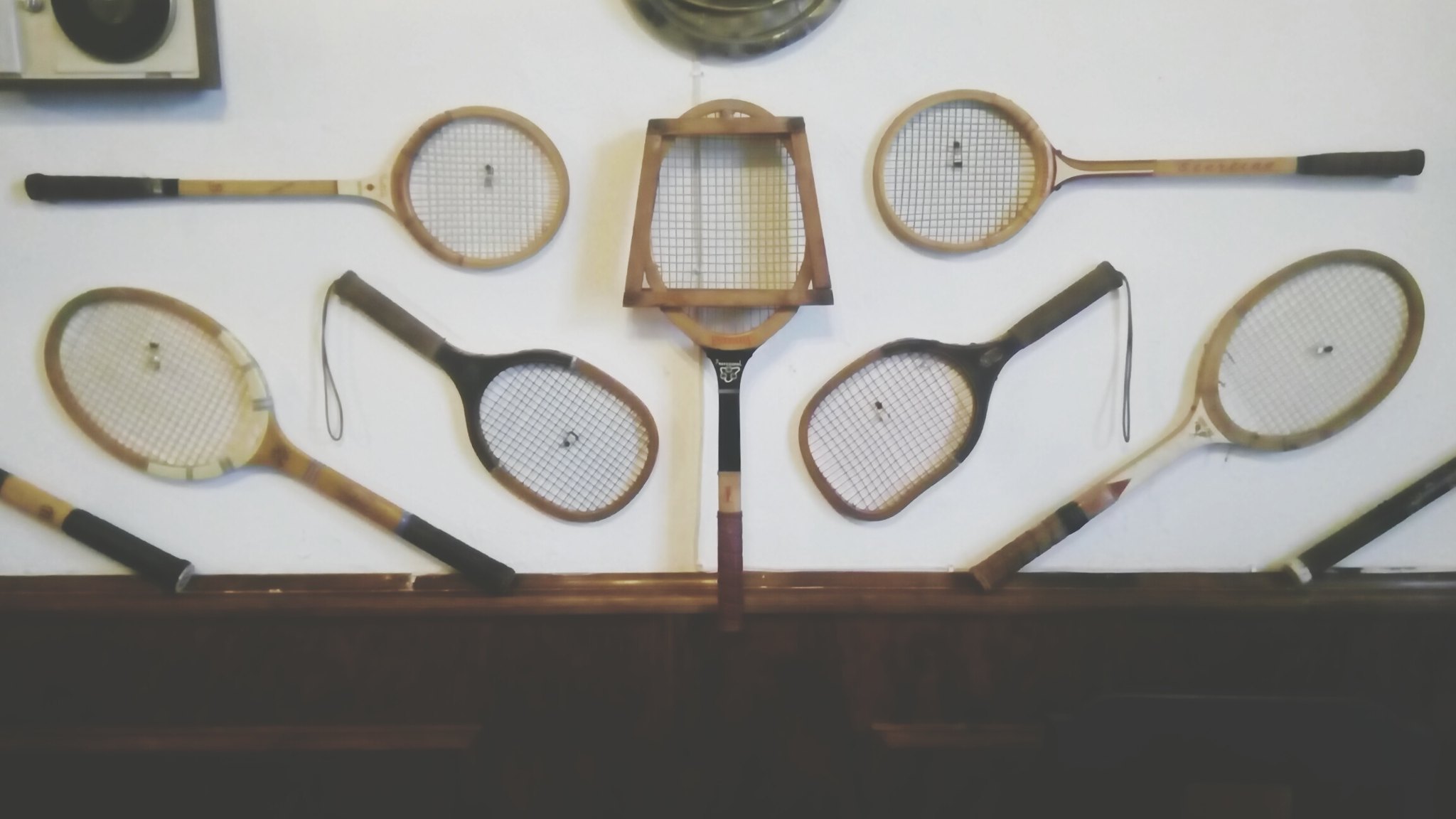The photograph captures a symmetrical display of various tennis rackets through the ages, all meticulously mounted on a white wall with a dark wood shelf below. In the center stands the largest racket, featuring a distinctive wooden frame that is trapezoidal in shape with an intricate netting design and a handle adorned in black, tan, and red hues. Surrounding this central piece are pairs of rackets, each mirroring its counterpart on the opposite side. To the right and left of the central racket are four tennis rackets, with one in each pair more oval and the other more rounded, and the smallest among them exhibiting a squarish frame. These rackets appear old and are crafted mainly from wood, with some featuring protective wooden frames on their hitting surfaces. The arrangement showcases an homage to the evolution of tennis rackets, with a couple even having hanging loops, possibly indicating some are for racquetball or badminton. Above the rackets, a partially visible object hints at further elements of the display, enriching the historical presentation.